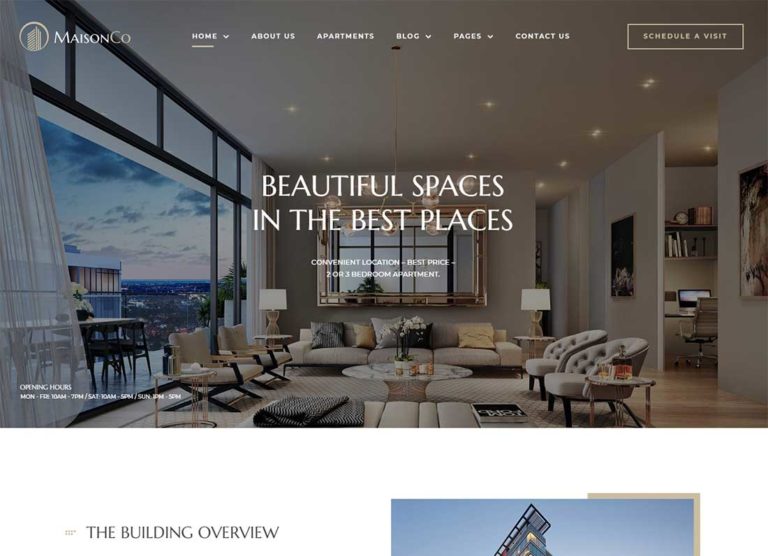The image showcases a high-floor apartment with an expansive city view. To the left, through a large window, a nearby skyscraper is visible with the bustling cityscape below and a serene body of water in the distance. The sky is partly cloudy, providing a tranquil backdrop.

In the top left corner of the composition, the logo of "Maison Company" is displayed atop an image of a building. The navigation menu spans across the top, featuring sections labeled: Home (underlined), About Us, Apartments, Blog, Pages, Contact Us, and Schedule a Tour, positioned in the top right corner. Dominating the center, the text reads "Beautiful Spaces in the Best Places" in large font, followed by "Convenient Location, Best Price, Two or Three Bedroom Apartment."

The main focus of the photo is the living area, furnished with a cozy couch adorned with numerous pillows, a large decorative mirror mounted above, and a coffee table accompanied by several chairs. To the right, there's a designated office space with a computer and a desk chair. Below the main text, the phrase "Building Overview" is mentioned, while the bottom right features a partial image of the sky and a fragment of a building.

The apartment's interior exudes elegance with its high ceilings and light-colored walls. A distinctive painting decorates one of the walls, adding an artistic touch. There’s also a small deck area visible outside the window, suggesting an inviting outdoor space. On either side of the couch are tables each topped with a lamp, contributing to the warm and inviting ambiance of the living area.